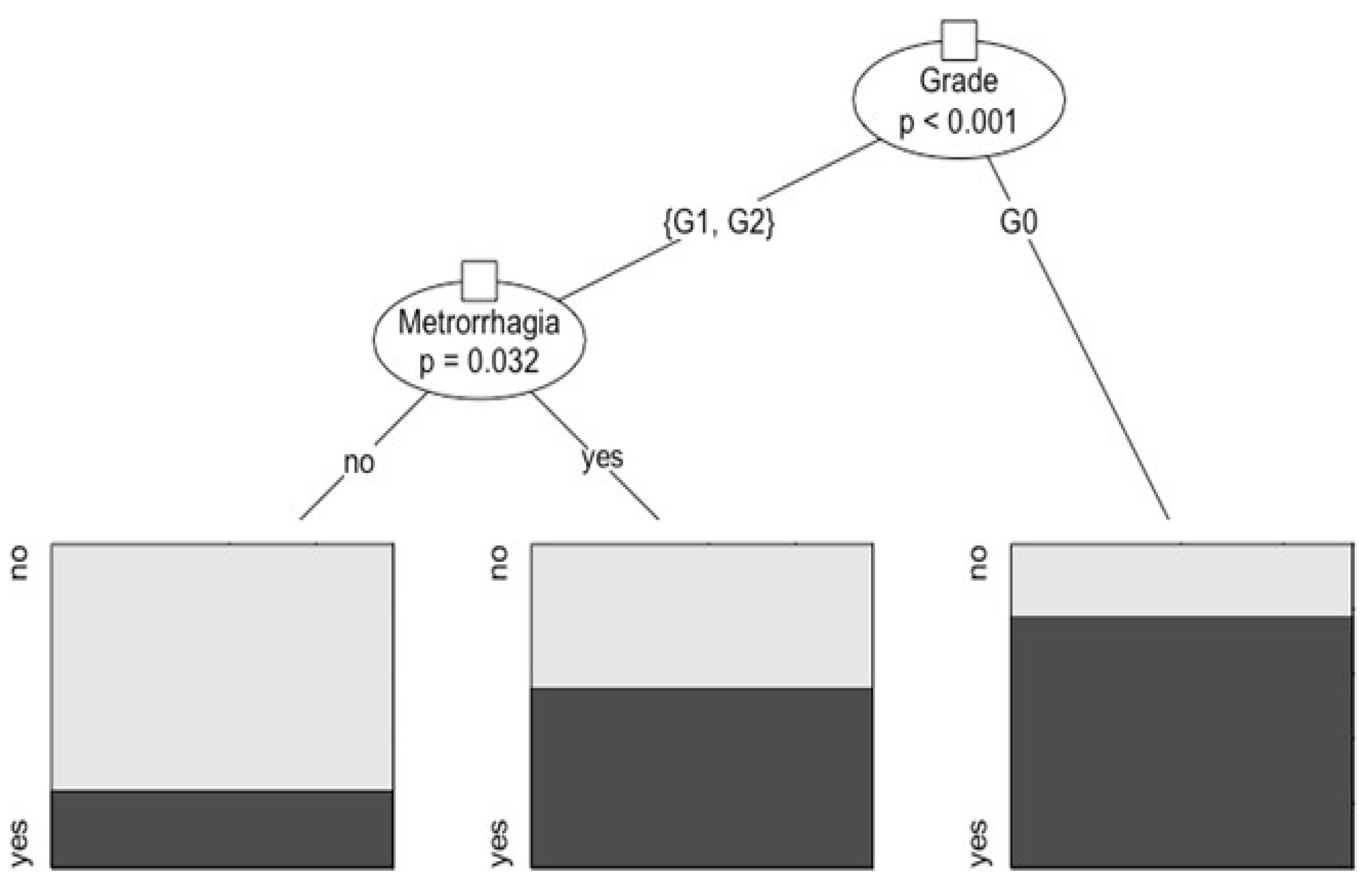The image depicts a detailed decision-making flowchart with a series of decisions represented through ovals and rectangles shaded in varying degrees to indicate proportions of outcomes. At the top of the diagram, an oval labeled "Grade, P < 0.001" directs to two lines. One line, labeled "G1, G2," leads directly to a decision box. This rectangular box has a small portion shaded in light gray labeled "No" and a larger portion shaded in dark gray labeled "Yes." 

Another line from the top oval extends to a second oval marked "Metro Regia, P = 0.032." This oval sends out two lines. The first line, labeled "Yes," points to a rectangular box shaded slightly more than half in dark gray (indicating "Yes") and just under half in light gray (indicating "No"). The second line from "Metro Regia," labeled "No," directs to another rectangular box. This box is predominantly shaded in light gray (indicating "No") with a smaller segment in dark gray (indicating "Yes"). 

The flowchart systematically illustrates how different grades and the condition of metro regia contribute to various decision points with proportional outcomes of "Yes" and "No."